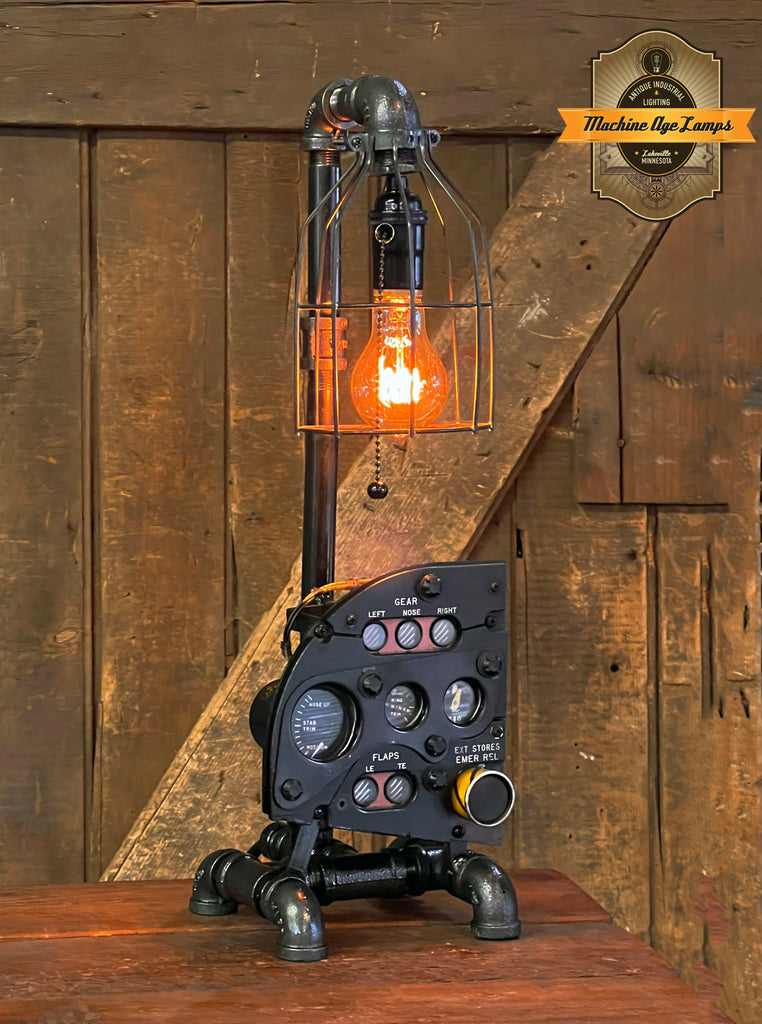The image depicts an intriguing lamp constructed from atypical materials, likely repurposed airplane parts, giving it a unique mechanical aesthetic. The base features a flat black panel adorned with various gauges labeled with terms like "gear," "flaps," "left," "nose," and "right," reinforcing its aviation origin. Supporting the lamp are rounded metal pipes that stabilize it on a wooden surface. Rising from the base, a metal pole extends upwards, bends at an elbow joint, and descends to suspend a large, glowing orange lightbulb. This lightbulb is encased in a protective metal cage and has a black base with a chain featuring a black ball hanging from it. The backdrop consists of rustic, medium-brown wooden planks, adding to the industrial vibe. In the top right corner, an overlaid graphic reads "Machine Age Lamps," labeling this inventive contraption as a lamp made from eclectic, vintage-inspired components.